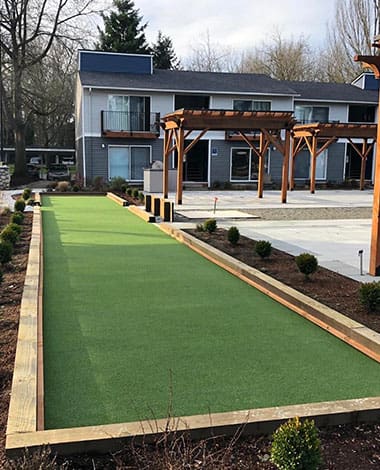This is a color photo taken outside during the day, capturing the detailed view of the backside of a two-story house set against a winter landscape. The house is painted in a sleek combination of dark gray and light gray. The backyard features a strikingly long strip of artificial green turf that resembles a mini golf course or putting green, framed by wooden beams and surrounded by beauty bark with small, decorative, green round plants.

To the left of the turf, an enormous tree towers over the scene, providing a significant contrast to the barren and evergreen trees visible above the house in the background. The right side of the yard is characterized by extensive concrete and tile work, interspersed with small bushes. A series of pergolas stand on cement slabs on this side, creating shaded areas ideal for lounging or picnicking. These structures extend slightly out of the photo's frame, suggesting there may be more pergolas just beyond the visible edge.